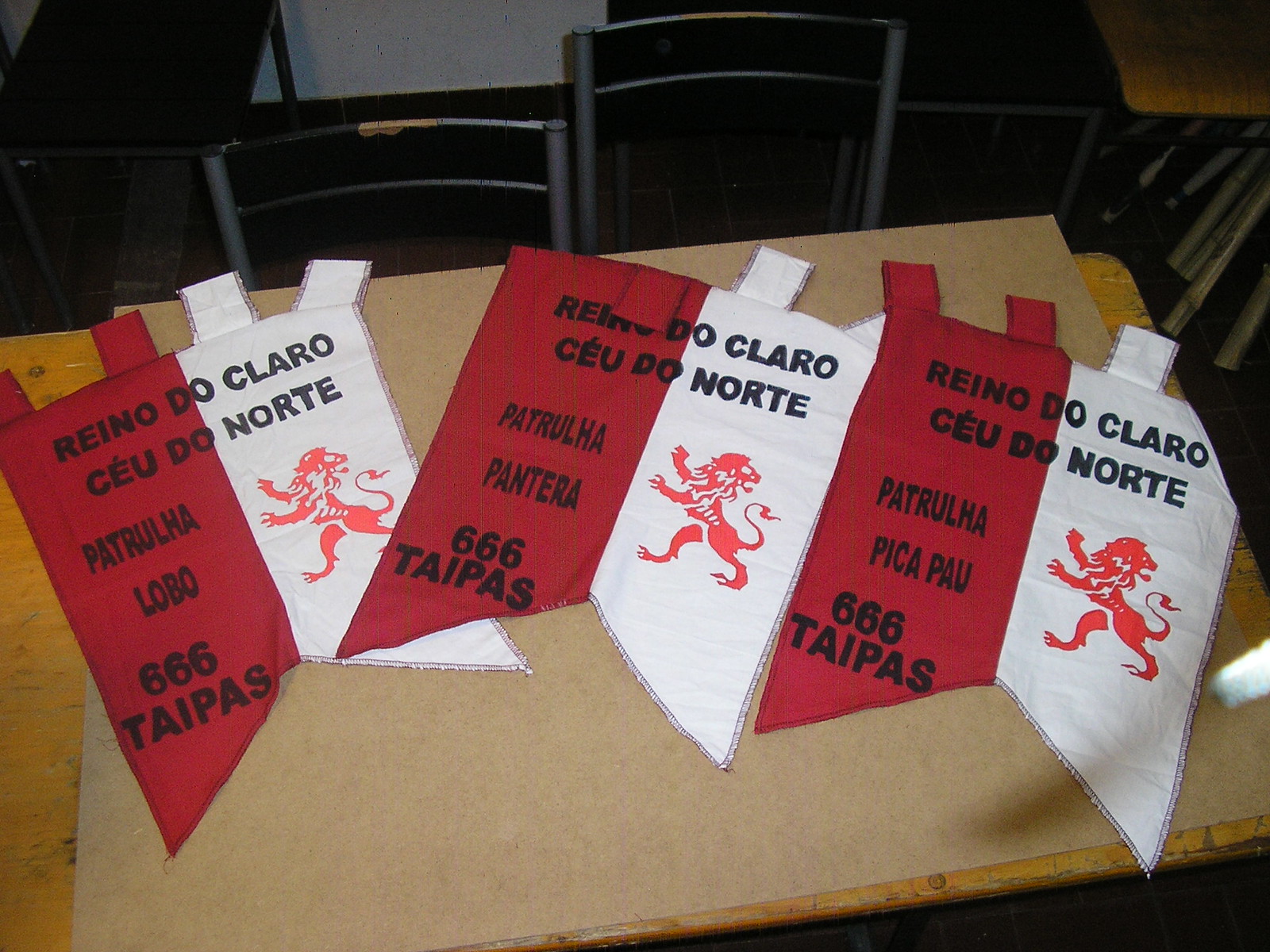In the photograph, taken at what appears to be a school desk with a laminate top framed by a wooden edge, three medieval-style banners are meticulously laid out in a row. Each banner is predominantly red on the left side and white on the right, and is adorned with a striking red lion emblem poised on two legs on the white section. The text on the banners seems to be in a foreign language, possibly Spanish or Portuguese, reading "Reino do Claro do Norte" at the top. Below this, the banners feature different inscriptions: "CEUDONORTA," "Pachacuma," "666 Tepaz," and "Lobo 666 Taipas." At the top of each banner, there are four hooks designed for hanging, likely intended to string them on a rod for display. The background of the image reveals a stack of various chairs, adding to the academic setting.